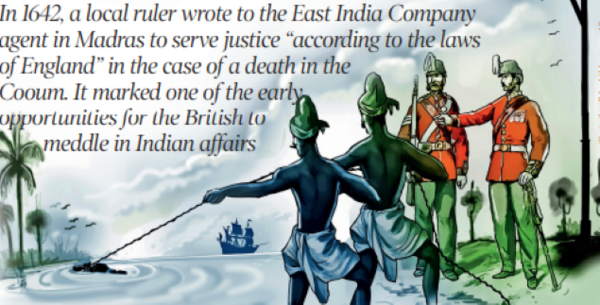An illustration from a historical book depicting an event in 1642, where British soldiers in red coats and green pants command two Aboriginal people, who are minimally clothed with towels around their waists and are shirtless. The Aboriginal people are pulling a body from a river using a rope, while the backdrop includes palm trees, birds flying, and a ship in the distance. The soldiers appear authoritative, emphasizing British intervention. At the top of the image, a caption reads: "In 1642, a local ruler wrote to the East India Company agent in Madras to serve justice according to the laws of England in the case of a death in the column. It marked one of the early opportunities for the British to meddle in Indian affairs." This scene highlights the early British influence in India, illustrating the cultural interaction and colonization dynamics of the period.